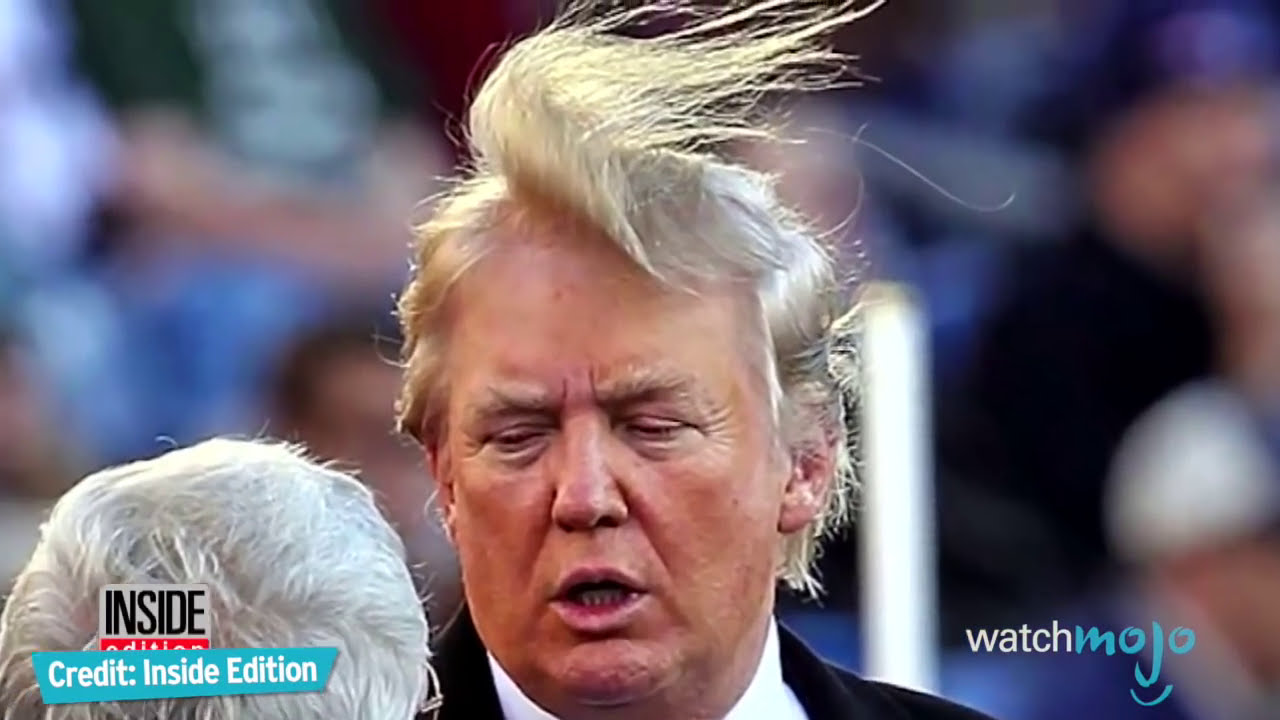This wide rectangular image appears to be a screenshot from a YouTube video or TV show featuring Donald Trump. Centered is Trump's head, characterized by his tan skin, squinting eyes, open mouth, and a concerned expression as he looks downward. His blonde hair, slightly lifted and wafting to the right, suggests windy conditions. In the blurred background, various people with light pink skin are seated, adorned in colors like black, light blue, green, red, and purple. In the top left corner, another person's head with gray hair is turned away from the camera. The bottom left corner of the image prominently displays two logos: "Watch Mojo," with "Watch" in white font and "Mojo" in blue brushstroke-style font, and "Inside Edition," which indicates the source of the image. The overall scene seems to capture a moment aimed at potentially amusing viewers by highlighting Trump's windswept hair and facial expression.